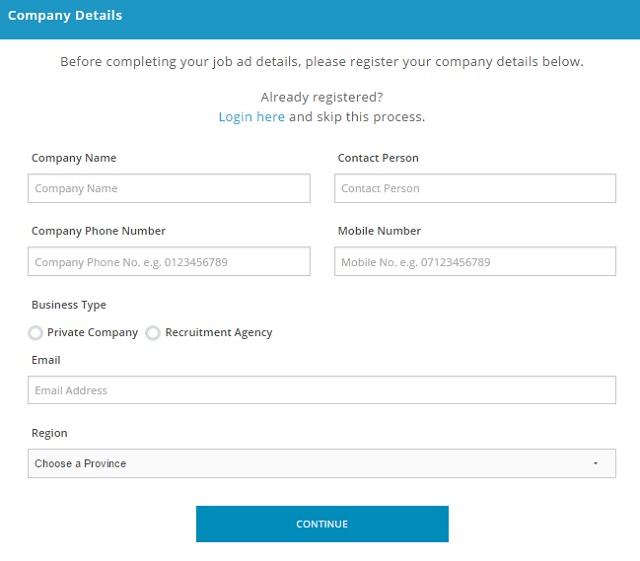**Detailed Description of the Online Form:**

The image showcases a screenshot of an online form, likely utilized as a template or example. Located at the top left corner is the heading "Company Details," clearly indicating the form's purpose. Directly beneath, there's an instructional text that asks users to "Please register your company details below before completing your job. Once you've registered, log in here to skip the process."

The form contains four primary fields for information entry, each distinctly labeled for clarity. These fields include:
1. Company Name
2. Contact Person
3. Company Phone Number
4. Mobile Number

Following these sections, the form requests additional information regarding the business type, providing options such as "Private Company" or "Recruitment Agency." Further, it asks for the company’s email address and region.

Positioned at the very bottom of the form is a prominent "Continue" button. This button is elongated and rectangular, colored in blue with the word "Continue" centered in white font, inviting users to proceed once all necessary information is provided. The entire form is set against a white background, maintaining a clean and straightforward design focused on user input.

In essence, this screenshot displays a structured and detailed online registration form intended for capturing essential company details before allowing access to further functionalities on the website.